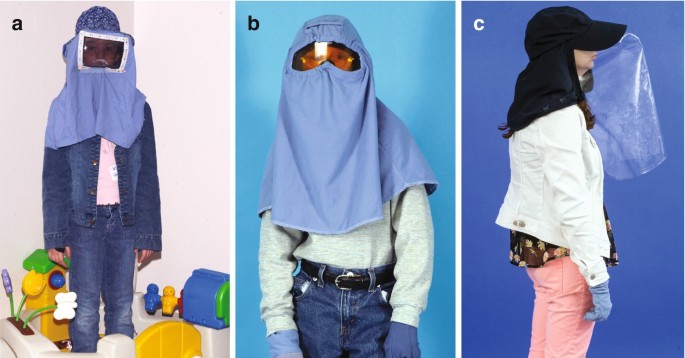The image consists of three different pictures, labeled A, B, and C, placed side-by-side, showcasing children wearing various head coverings and safety masks. In Picture A, located on the left, a child is dressed in a blue jeans and jacket ensemble with a white shirt underneath. The child also wears a blue headdress resembling a beekeeping mask or safety helmet that covers the head and face down to the shoulders. The image includes children's toys scattered around the child's feet. Picture B, in the center, features another child dressed in denim jeans and a gray sweatshirt, wearing a blue head covering similar to a hood. This covering includes yellowish-amber goggles integrated into the headgear, allowing the child to see out. Finally, Picture C, on the right, shows a girl wearing a white jacket, pink jeans, and gloves. She is dressed in a black hat with an extended cover that goes down to her shoulders, paired with a large, clear plastic shield hanging in front of her face. The overall theme of the images suggests that these head coverings and masks are designed for safety, possibly to protect against germs or insects.